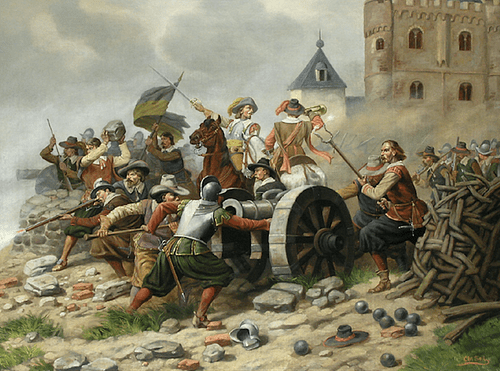The image depicted is a historical painting of a dramatic Middle Ages battle scene, set in front of a towering, tan castle with a distinct gray and white steeple. The battlefield is chaotic, with figures actively engaged in the thick of combat. Men dressed in elaborate, blousy shirts, reminiscent of Dutch master styles, and adorned with pirate-like hats and metal helmets are prominent. There are also warriors in metal-looking vests and sashes, some wielding swords, others aiming guns or using long sticks to load cannonballs into massive cannons, which have large round wheels and metallic hues. One distinctive figure on horseback holds a sword, seemingly ready to charge down a mountain, while others either carry supplies or aim their weapons. The ground is littered with cannonballs and discarded hats, underscoring the intensity of the skirmish. The painting features a smoky, gray sky, implying the aftermath of cannon fire, and the scene fades into what could be mountains or water, adding depth to the background. The overall impression is one of a tumultuous and vividly detailed portrayal of an ancient battle, possibly a period piece displayed in a museum or an art gallery.